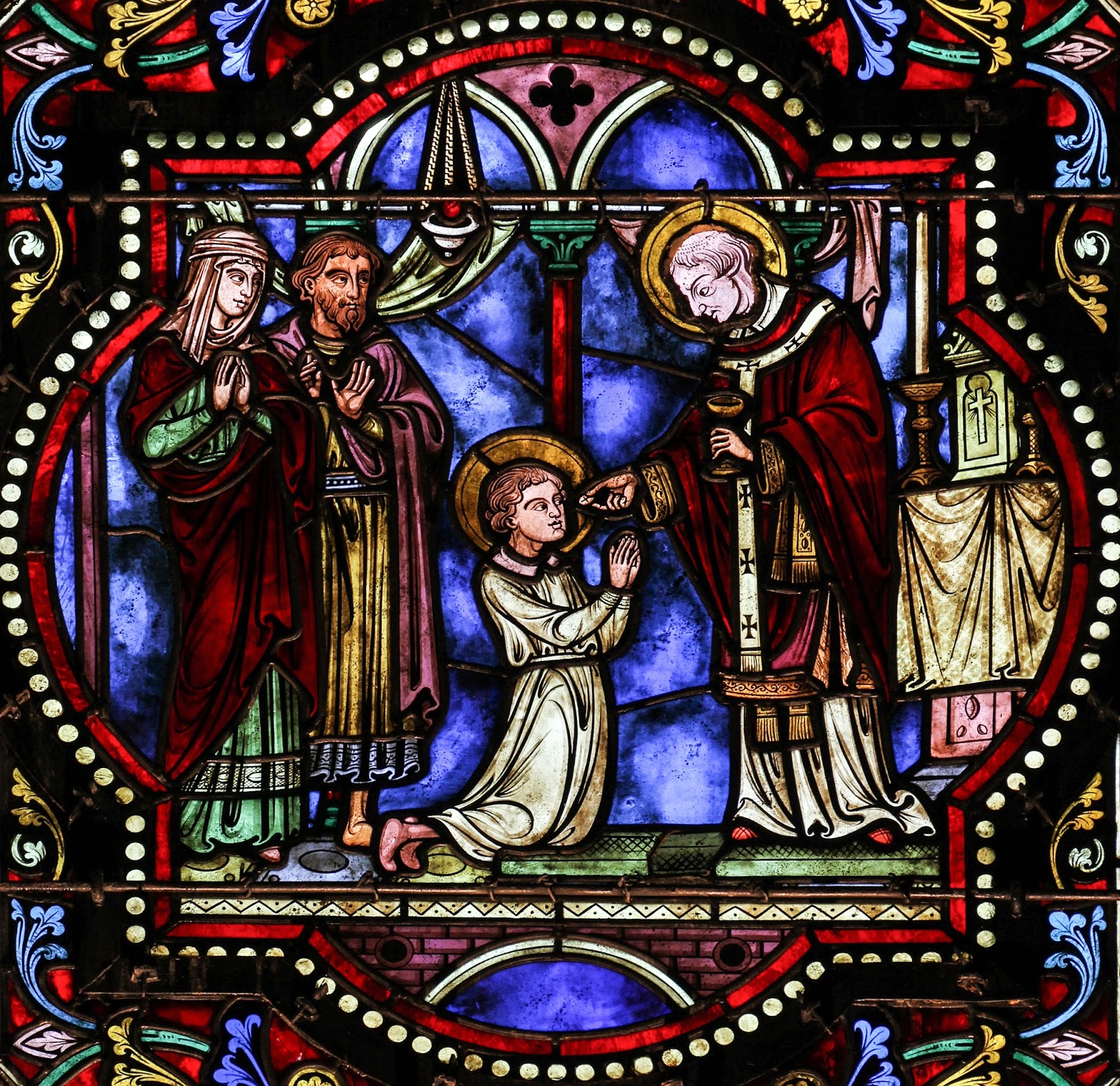The stained glass artwork depicts a religious scene reminiscent of Catholic traditions, capturing a moment of solemnity and reverence. Central to the image is a small child, dressed in a white robe, kneeling and receiving communion from a priest adorned in a dark red robe with a golden halo. The priest's hand extends toward the child, offering a host while holding a wooden chalice. The vivid colors of the glass mural include shades of blue, red, white, brown, purple, and gold, enhancing the scene's sacred ambiance. Flanking the child are two figures, a man and a woman, likely the child's parents, exuding joy and devotion, dressed in long, colorful robes in hues of burgundy, light purple, gold, and green. The woman wears a distinct white head accessory. In the background, an altar with lit candles and a hanging incense burner completes this deeply spiritual tableau, suggesting the child's first communion and his parents' celebration of this significant rite of passage.